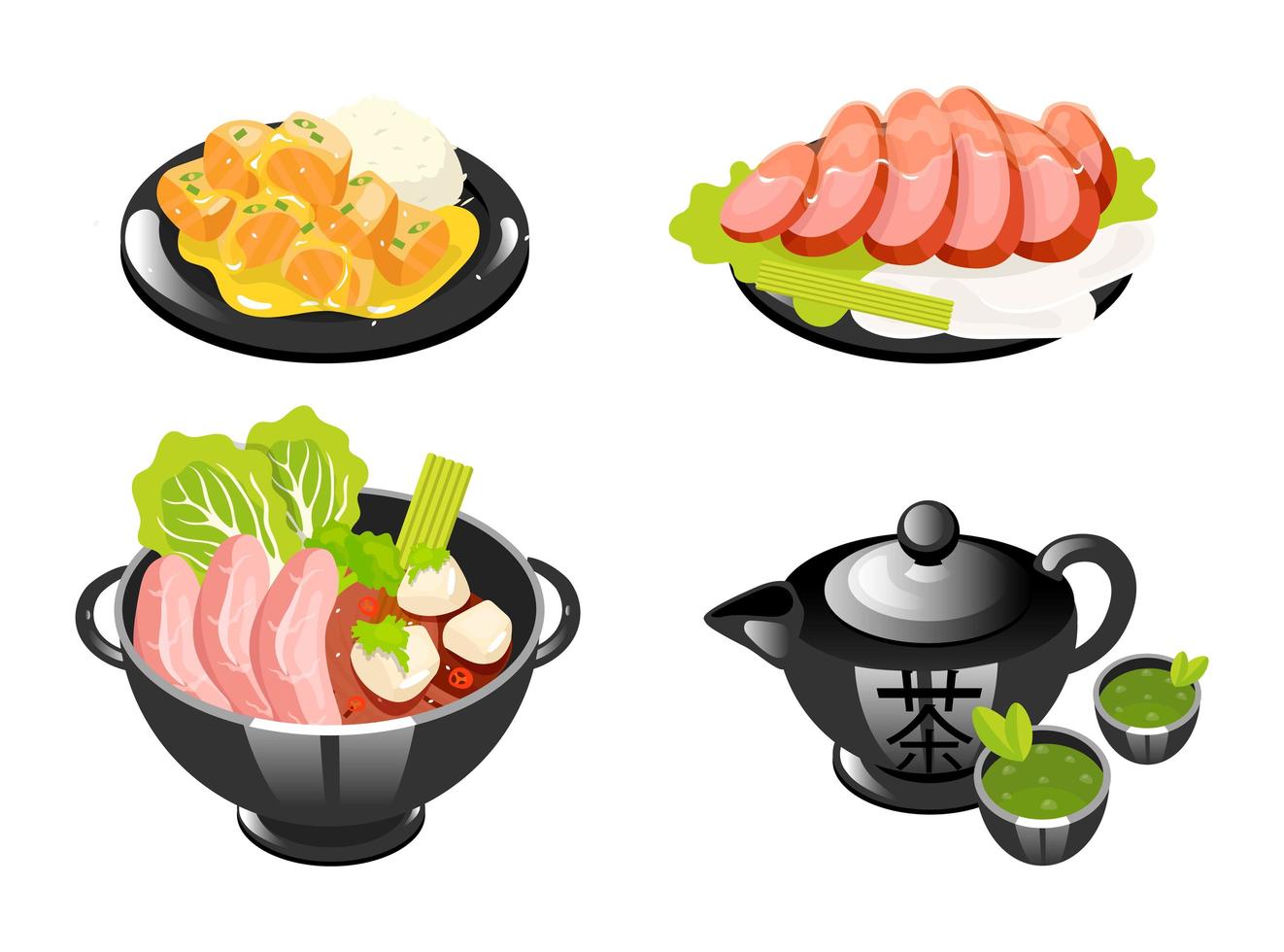The image is a cartoony illustration resembling clipart, featuring four different depictions of Asian dishes on a white background. In the top left, there is an intricate black plate holding a white rice ball alongside pieces of orange chicken adorned with tiny green spices or green onion. On the top right, another black plate contains slices of pink raw fish atop a large green leaf, accompanied by white rice. The bottom left showcases a black colander-style bowl with handles, filled with a medley of green cabbage, chunks of pink fish, white balls, green broccoli leaves, and possibly sprigs of parsley. Finally, on the bottom right, there is a black teapot featuring Asian lettering, flanked by two black teacups containing green tea with small green leaves. The overall style of the artwork is simple yet detailed, providing a charming and illustrative representation of various Asian culinary delights.